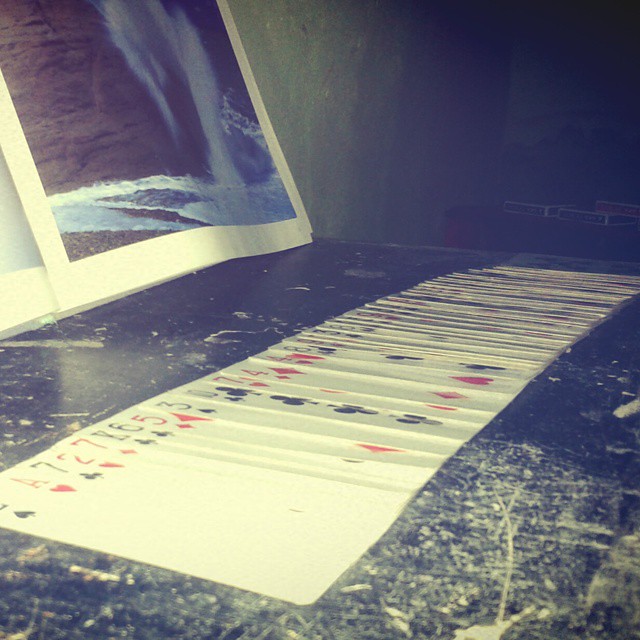The image showcases a collection of playing cards neatly arranged side-by-side, although slightly overlapping, stretching from the lower left of the image to the middle right. The cards are laid out on a black granite table speckled with white. The photograph appears somewhat overexposed, casting a bright sheen over the scene. In the top left corner, a magazine featuring an image of a waterfall on the visible right page lies partially within the frame, with its left side cut off. Behind the table and magazine, a plain, slightly dark green wall serves as the backdrop. In the middle top right of the image, a few boxes of playing cards are visible, with two navy blue boxes and one red box completing the composition.